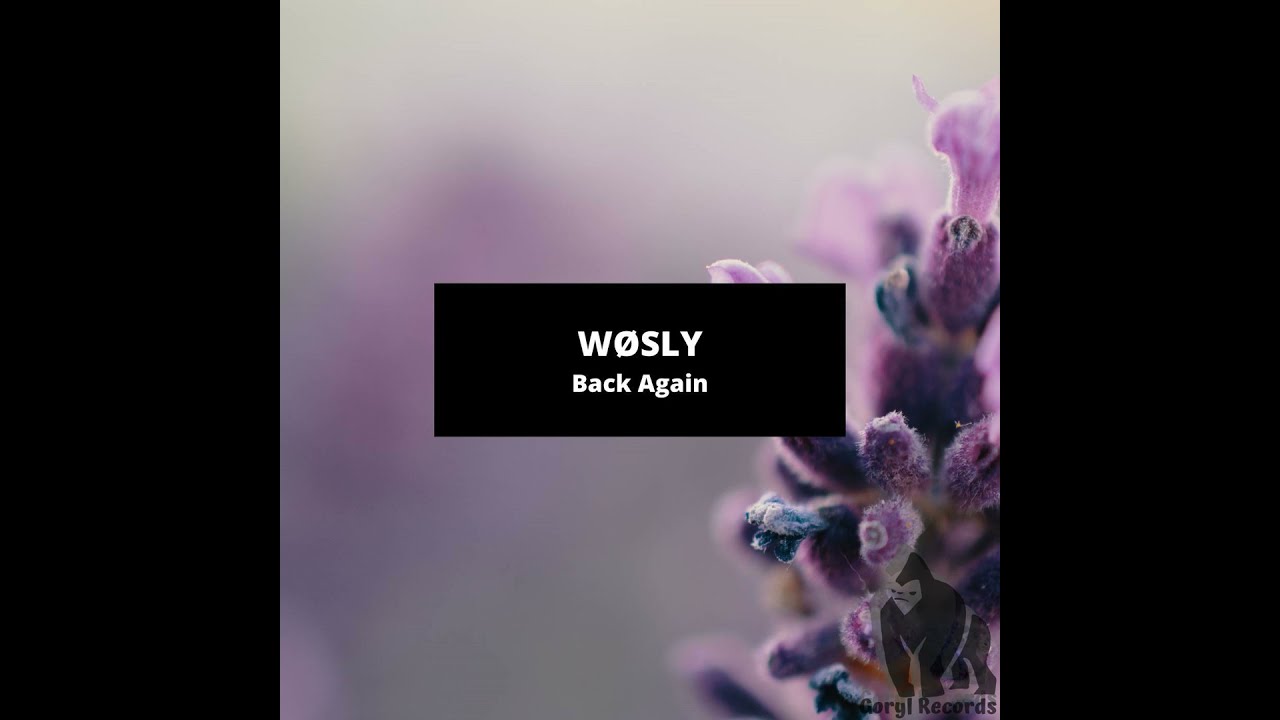This image features a central black rectangle with white text that reads, "WOSLEY back again," with the 'O' in WOSLEY having a line through it. The image is bordered by two thick black vertical strips on the left and right sides. Dominating the scene is a vibrant purple sea creature, adorned with blue and orange hues, resembling an underwater entity. This creature, positioned slightly to the right, has an intricate structure with multiple protrusions akin to a unique flower rather than traditional petals. The background is a blurred underwater environment with hints of additional purple forms, possibly other similar creatures or flowers. In the bottom right corner, there is a graphic of a gorilla standing on its front legs, adjacent to text that might read "GORAL RECORDS." The main creature in the foreground is clear and detailed, while the background remains obscure and fuzzy, emphasizing the depth and dynamic nature of the underwater scene.